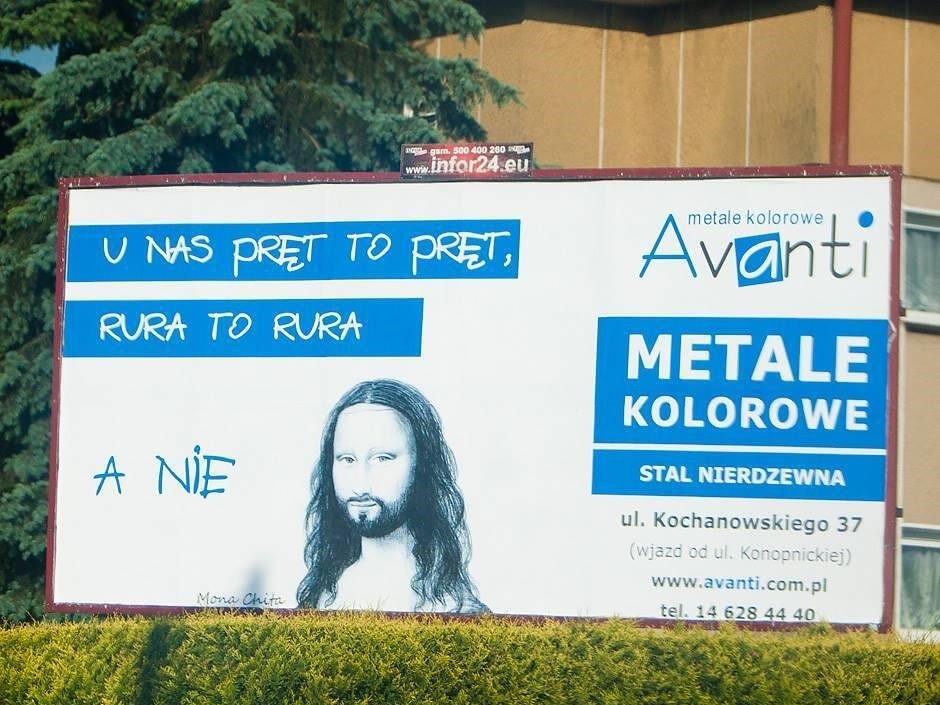The image is an outdoor advertising board framed in brown paint, noticeably marked with several white spots from bird droppings on the top. Placed beside a brown building and a conifer tree with light green hedges growing below, the board primarily showcases a white background with sections of blue. Starting from the top left corner, the board features blue rectangular banners that sequentially read "U-N-A-S-P-R-E-T-T-O-P-R-E-T" and "R-U-R-A-T-O-R-U-R-A." Centered below these banners is a hand-drawn image of a smiling man with a mustache, beard, and long hair, resembling a male version of the Mona Lisa. To the right of this image, in cursive text, it reads "Mona Chita," and to the left, the letters "A-N-I-E" appear in blue text. Further details include repeated entries of the phrases "Metale kolorowe" and "Avanti," along with additional information: "Stal, Nied zevna, ul.koczernowskiego, 37, Wejazd od U, Konop Nikolaj, www.avanti.com.pl," and the telephone number "146284440."